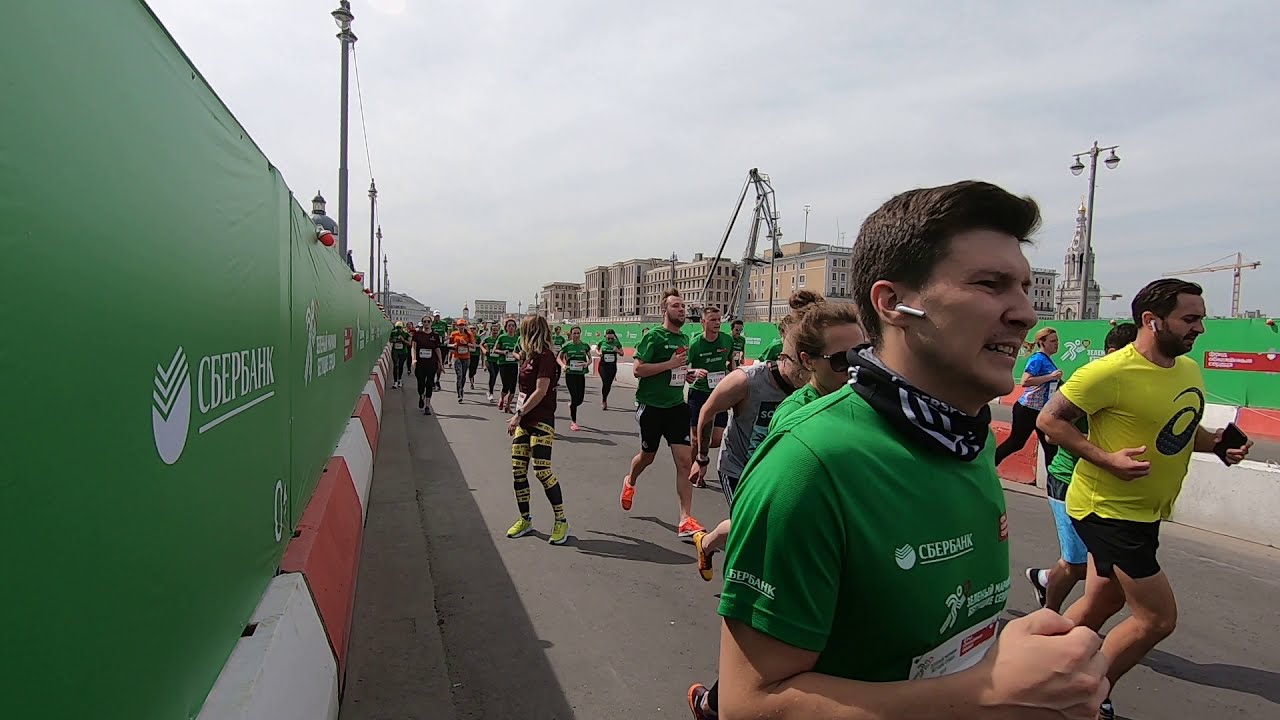In this vibrant city scene, a foot race is underway with the majority of participants wearing green t-shirts, likely the event's official attire, each one labeled with numbers or stickers indicating their registration. The race is taking place on a paved asphalt street bordered by red and white barriers and green fencing, which might feature writing in what appears to be a European language, possibly Russian. The runners are moving towards the camera, but not directly at it, and form a line that recedes into the distance.

At the forefront, a man in a green t-shirt stands out with his short brown hair, smiling face, and Apple earpods. He also wears a blue and white scarf around his neck. To his right, another man in a yellow t-shirt with a black logo, black shorts, dark hair, a beard, and holding a phone in his left hand is also running with ear pods in his ears. Nearby, a woman with shoulder-length blonde hair, dressed in a dark t-shirt and gold and black jogging pants, has paused and is looking behind her.

The backdrop consists of urban buildings and city lights, with construction cranes visible, indicating ongoing development. The sky is somewhat cloudy but patches of sunlight peek through, adding a contrasting brightness to the scene. The view encapsulates the essence of a well-organized, spirited race, possibly for charity or as a community fun run, against the vivid backdrop of a city bustling with life and energy.